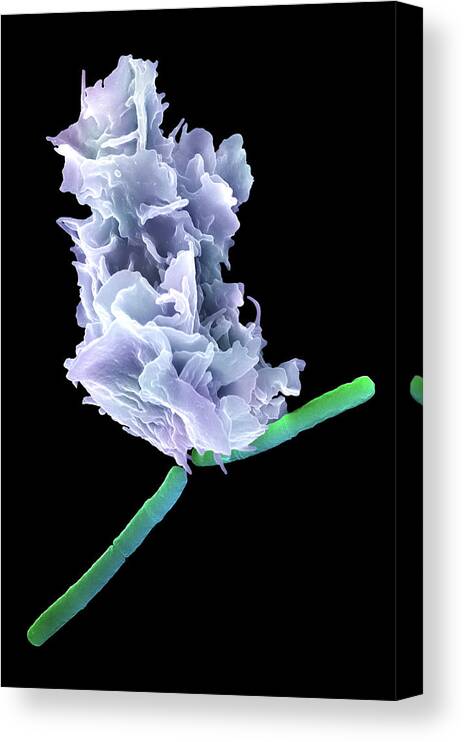This image captures a vertically oriented rectangular object set against a plain background. The object is entirely black and positioned at a slight angle, which reveals a subtle depth on its right side, giving it a three-dimensional appearance. The surface of the object is adorned with two green, stem-like elements. Positioned atop these stems are intricately ruffled structures, which exhibit a light lavender to purple hue. The ruffled formations rise upward, adding an element of delicate texture to the scene. The exact nature of these ruffled structures is ambiguous, though they evoke a floral resemblance. A small segment of the green stem-like part is also visible on the right side, contributing to the organic look of the entire composition.